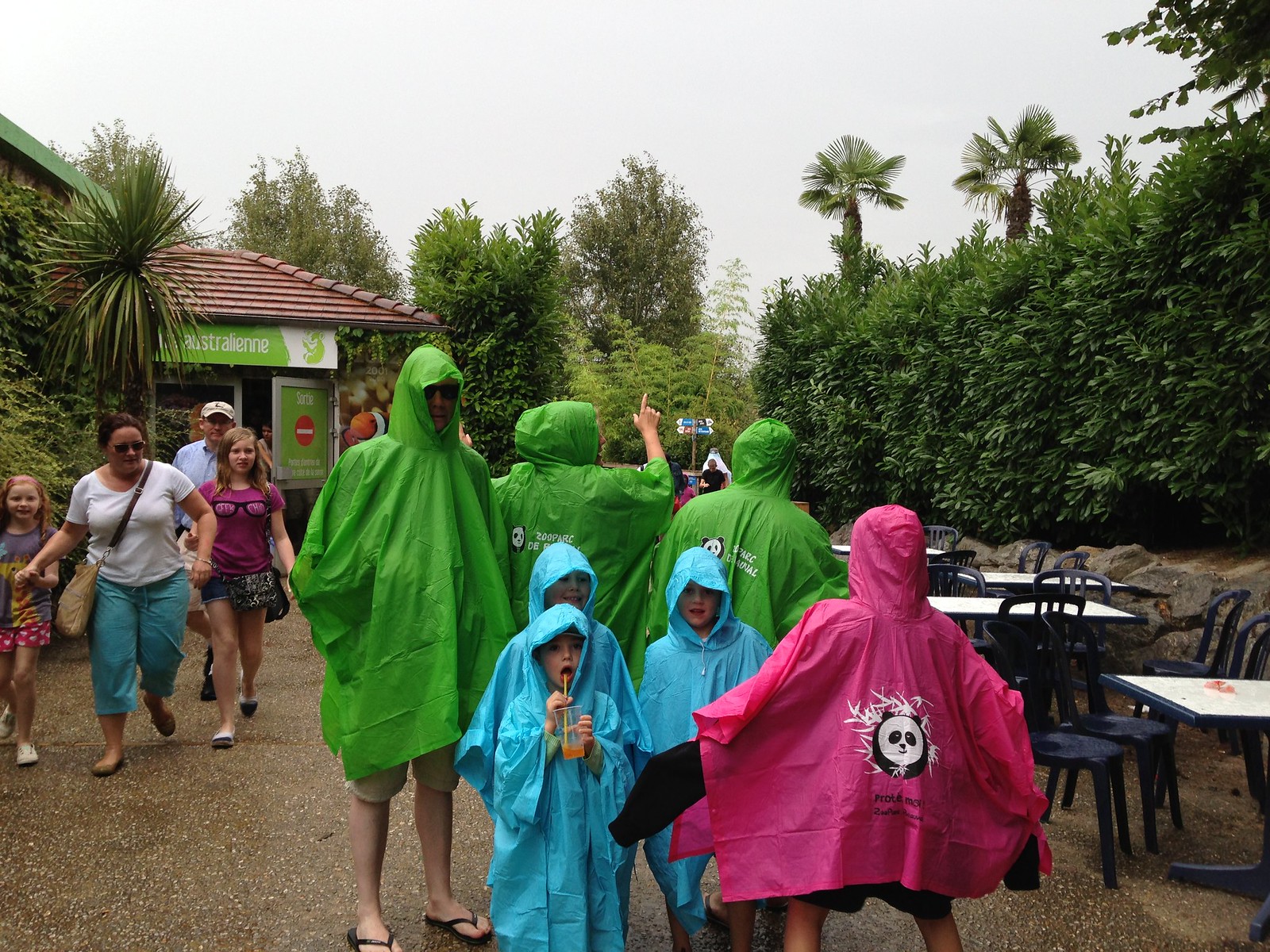In this photograph, taken at an outdoor adventure park or zoo on a wet, gray overcast day, the foreground features a family of seven people. Three adults wear green ponchos, and three young children are in blue ponchos, with one preteen off to the right in a red poncho with a panda on the back, displaying the "Zoo Park" logo. Surrounding them, the background reveals a gravel pathway flanked by tall palm trees and lush, bushy greenery. To the right, black and white tables are arranged, likely for eating snacks. A series of directional signs and a tent showcasing animal information, featuring pictures of a koala and a clownfish, can be seen towards the center-right. On the left-hand side, another family of four—two parents and two girls in shorts—not wearing ponchos, appear to be walking towards the viewer, hurriedly escaping the rain. The area’s design, with its natural yet structured layout, mimics that of typical zoo settings.